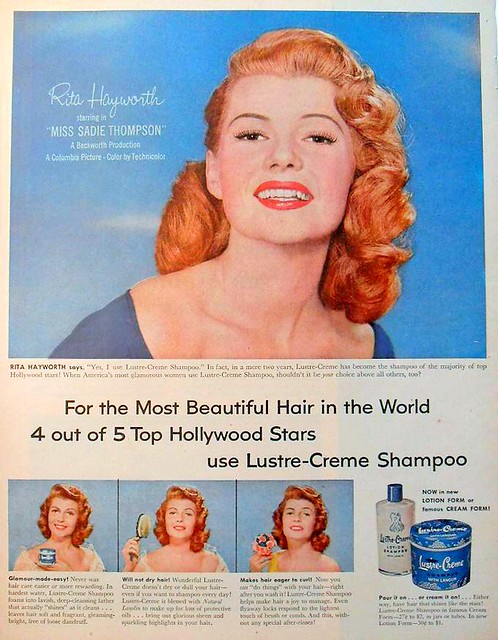This is a full-page vintage magazine advertisement, likely from the 1940s, for Luster Cream Shampoo. At the very top, there is a prominent, smiling photograph of the famous actress Rita Hayworth, who has striking red hair and is directly engaging with the camera. The text around her photo reads: "Rita Hayworth starring in Miss Sadie Thompson, a Columbia picture, color by Technicolor." Below the main photo, an advertisement slogan declares, "For the most beautiful hair in the world, four out of five Hollywood stars use Luster Cream Shampoo." 

Further down, the ad features three smaller images of Rita Hayworth. In the first, she is holding a jar of Luster Cream Shampoo. In the second, she is holding a brush, and in the third, possibly a mirror or another grooming item. Each image is accompanied by a paragraph of text that's too minute to decipher. Lastly, in the lower right-hand corner, the ad showcases both a jar and a tube of Luster Cream Shampoo, with additional text detailing the product benefits, although this text is also too small to read clearly.